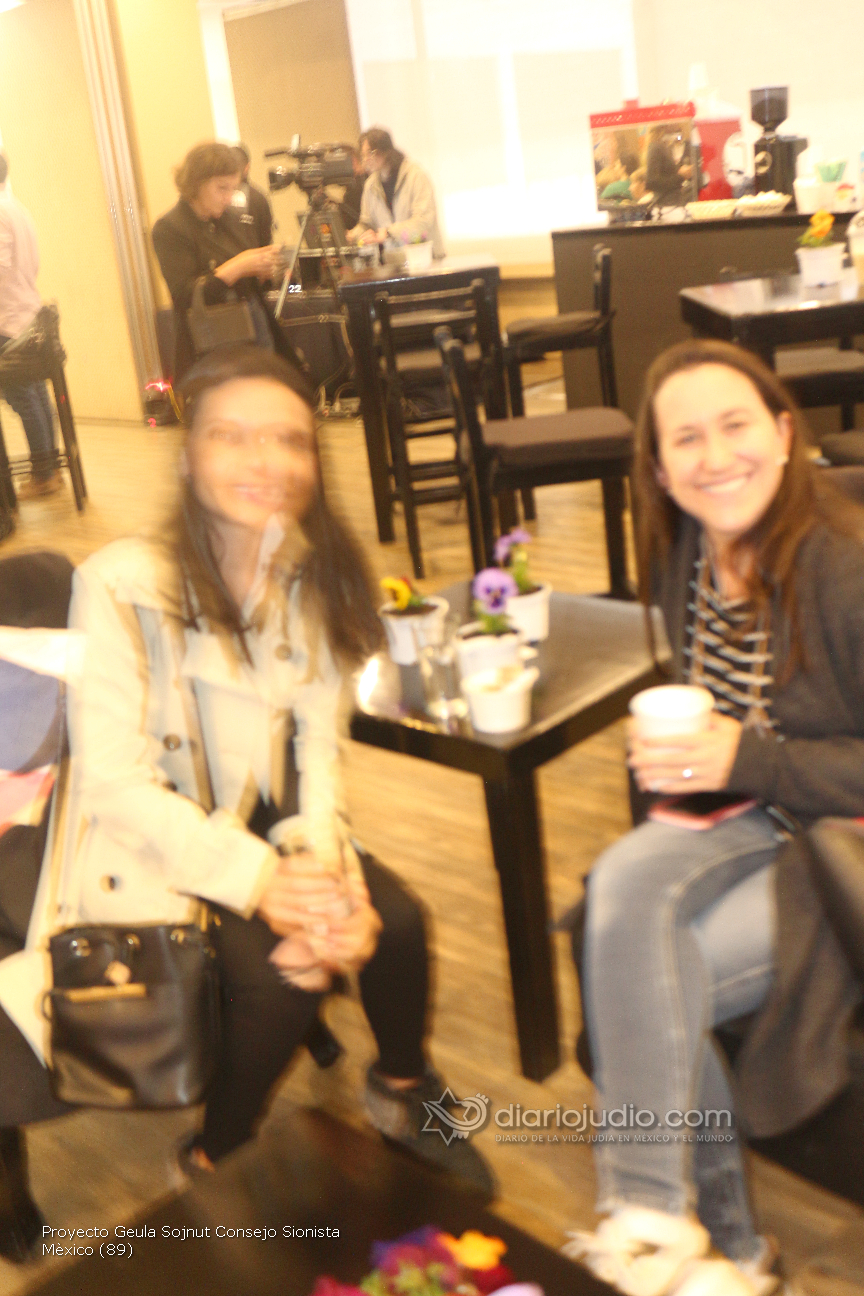The image depicts two women sitting at a square black table in a bustling coffee shop, both dressed in jackets and smiling at the camera. The woman on the right is more in focus, with red hair, wearing denim blue jeans, a gray sweater, and a black-and-white striped top. She’s holding a white coffee cup. The woman on the left is quite blurry, possibly due to movement; she has dark hair, a white sweater, black pants, and a bag hanging on her shoulder. Both women have their legs crossed. The table they share has small pots with sunflowers and purple flowers in white containers. Visible in the bottom left of the photo are the words "PROYECTO GEULA SOJNU T CON SEJO SIONISTA Mexico (89)," alongside a watermark that reads "DiarioJudio.com" with a small star and logo. The background reveals a lively scene with a variety of black tables, some adorned with similar flower arrangements, and other patrons, including a woman on her phone with a purse hanging to her side. Additionally, there is a person operating a large video camera setup in the upper left corner near a desk area.